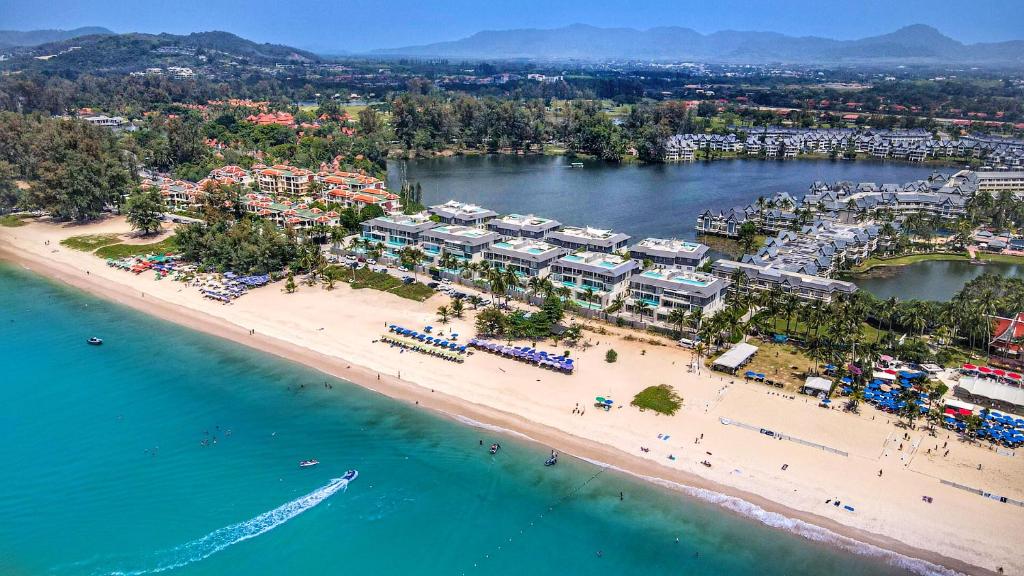This image is an overhead aerial shot of a captivating coastal area featuring a sandy beach strip surrounded by water on both sides. The front side of the strip meets the ocean, where boats and people can be seen, with waves gently lapping against the shoreline. The opposite side resembles a lake, characterized by blue waters. Lining the sandy shore, there are rows of neatly arranged blue chaise lounges and umbrellas, adding to the serene atmosphere.

Behind the beach, there is a cluster of multi-storied blue buildings that could be either homes or hotels, constructed in a similar architectural style. Further back from these structures, the image reveals a small greenish lake or pond. To the left, the scene transitions into a larger blue lake bordered by a coast of white cliffs and surrounded by lush green trees.

In the lower left corner of the image, a blue lake stands out with a boat floating in its center. Adjacent to this lake is the sandy beach with its array of chairs. To the right, additional buildings with red roofs are visible, and the left part of the landscape showcases some hills, with more distant and faint hills visible towards the right. Altogether, this detailed image portrays a picturesque and dynamic coastal landscape.